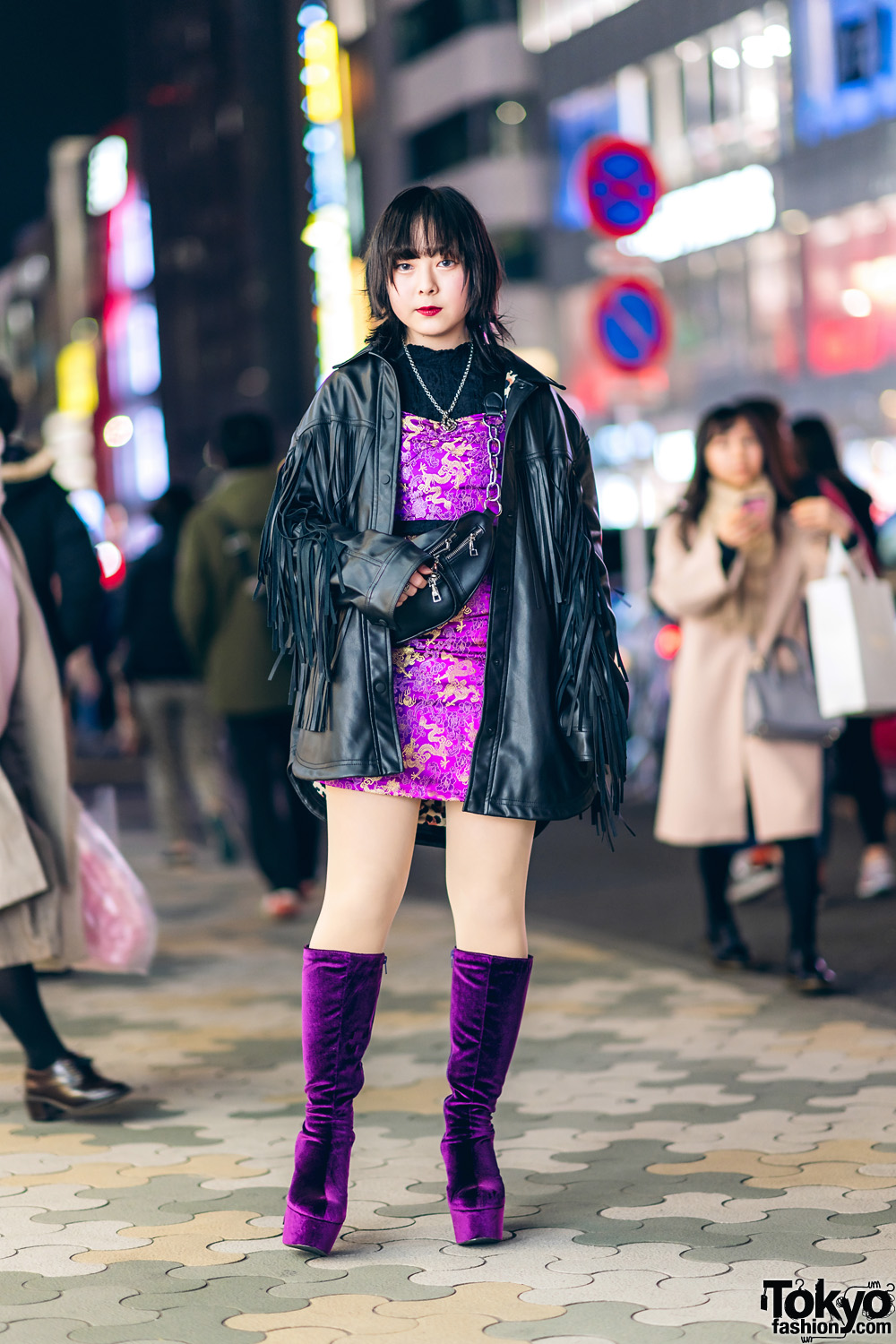This photograph showcases a fashionable young Asian woman standing prominently on a vibrant city street at night. She wears striking purple suede knee-high boots and a matching purple mini dress adorned with gold dragons. Her outfit is complemented by a fringed leather jacket of the same length as the dress and a leather purse, which she clutches. Her accessories include a metal chain necklace, and she is styled with an eye-catching bob haircut with bangs and vibrant red lipstick. The background captures the bustling city atmosphere with blurred pedestrians and buildings illuminated by neon lights. The ground beneath her feet is a patchwork of gray, yellow, and green stone tiles. The image is branded in the bottom right corner with the label "TokyoFashion.com."